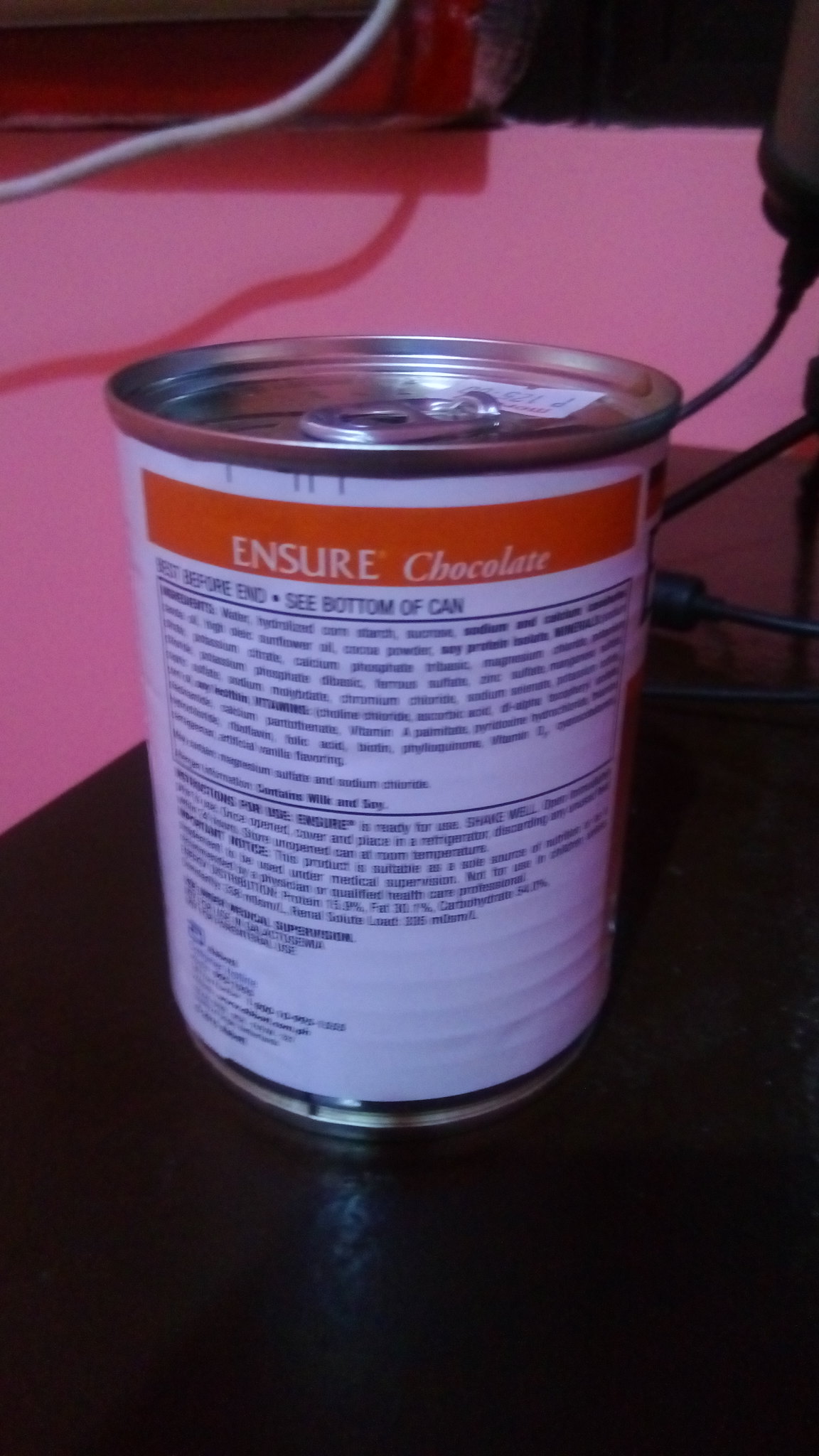This image features a close-up of an unopened Ensure chocolate flavor meal replacement drink can. The can's visible side showcases an orange banner with the words "Ensure Chocolate." Below this banner, the rest of the can's exterior is white with black lettering. Key phrases are legible, such as "Best before end, see bottom of can." The can includes detailed information about the product, including an ingredients list with approximately eight to nine lines. Additional text mentions an important notice, the company name, address, manufacturing address, and phone number. This silver can has a flip-top lid and sits on a black or ebony nightstand or table. The background features pink walls, and an array of cables, including a white cord at the top and several black cords on the right, along with a partially visible brown box with a cord emerging from it.